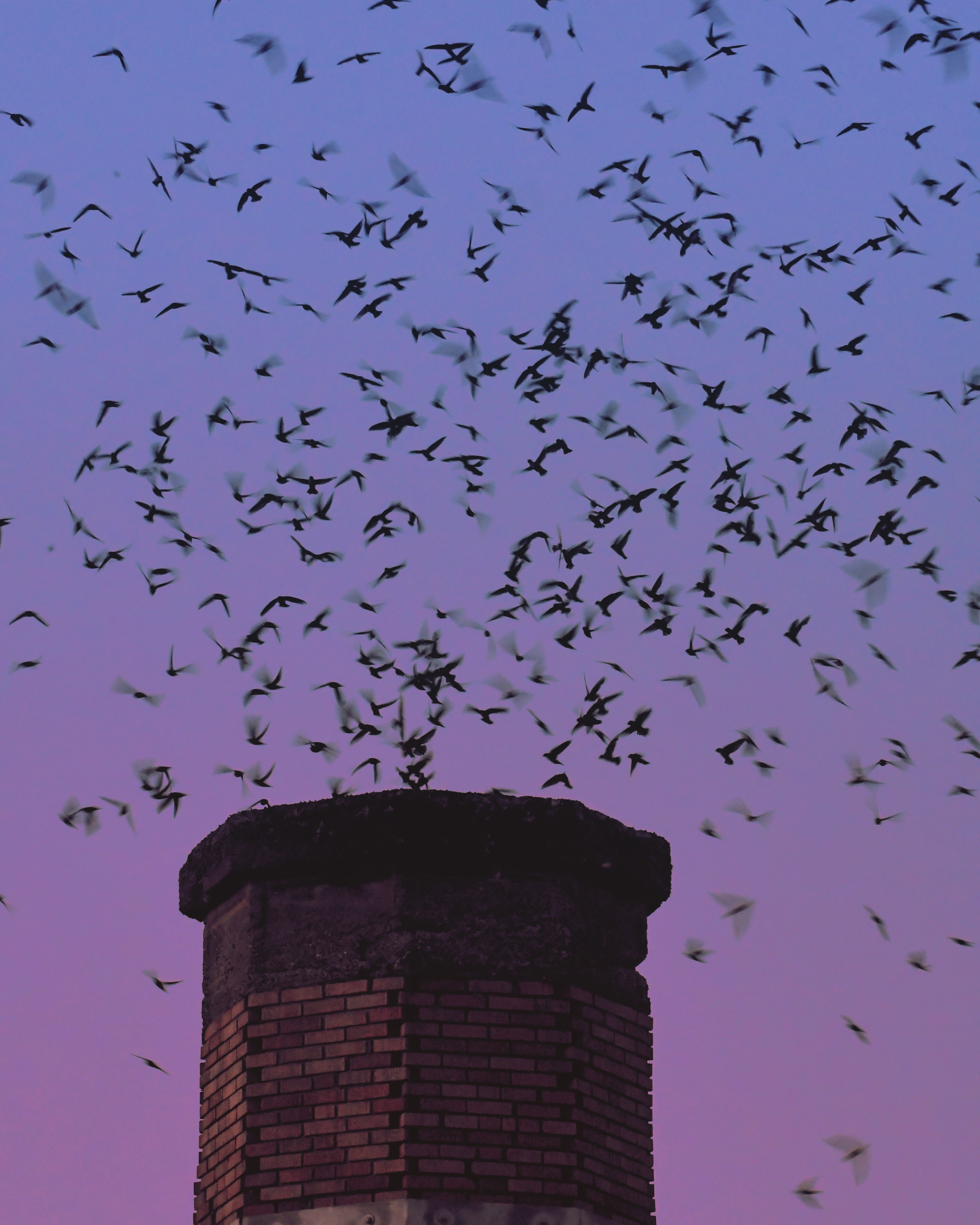The photograph captures an enchanting scene during sunset, characterized by a backdrop of a subtly fading sky transitioning from deep dark purple to a lighter lavender hue, eventually becoming a soft blue. Dominating the bottom portion of the image is a prominent masonry structure, possibly a large chimney stack with a unique polygonal shape, likely pentagonal or hexagonal, built from red-orange bricks.

Encircling the structure and scattered across the sky are hundreds of birds, depicted mostly in sharp silhouette against the vibrant twilight. The sheer number of birds, possibly numbering in the low hundreds, are distributed throughout the photo with varying degrees of clarity—some are beautifully sharp, while others appear blurred, emphasizing their dynamic flight. The scene evokes a mesmerizing interplay between the orderly architecture of the brick chimney and the chaotic swirl of avian silhouettes against the serene, colorful twilight sky.